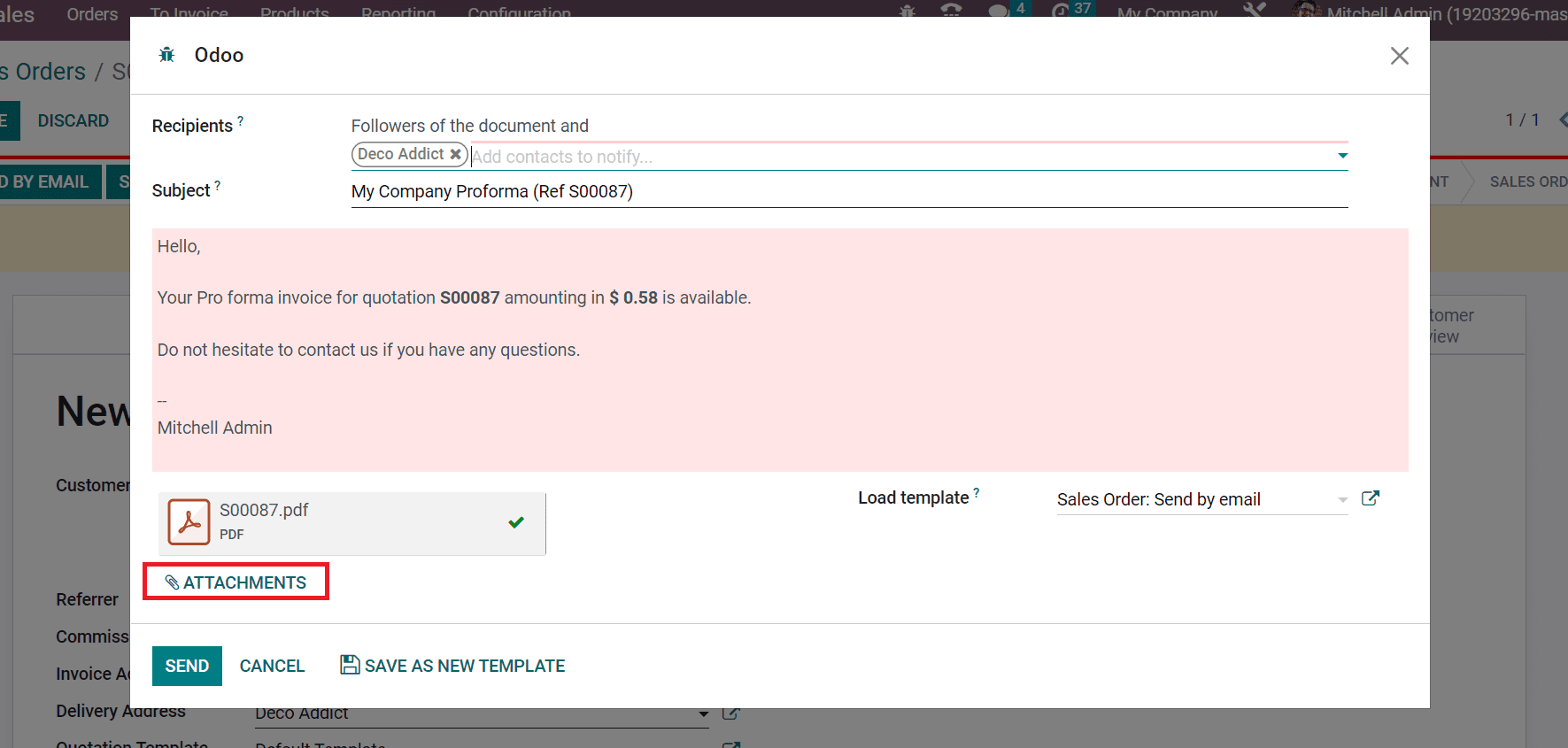The image features a pop-up window on a white background with black lines, displaying details of an invoice document. The top of the window includes fields labeled "ODO," "Recipients," "Followers of this Document," and "DECO." The subject line reads "My Company, ProPharma," with a reference number "S0087."

In the center of the pop-up, a pink shadow box contains a notification stating: "Hello, your ProPharma invoice for quotation S0087 amounting to $0.58 is now available. Do not hesitate to contact us for any questions." Below this message, the sender's designation is listed as "Provincial Admin."

At the bottom of the window, there is a highlighted "Send" button along with additional options for "Cancel" and "Save as a New Template." A PDF attachment is also indicated within this section. The background behind the pop-up window appears indistinct, suggesting it is related to the invoice creation process.